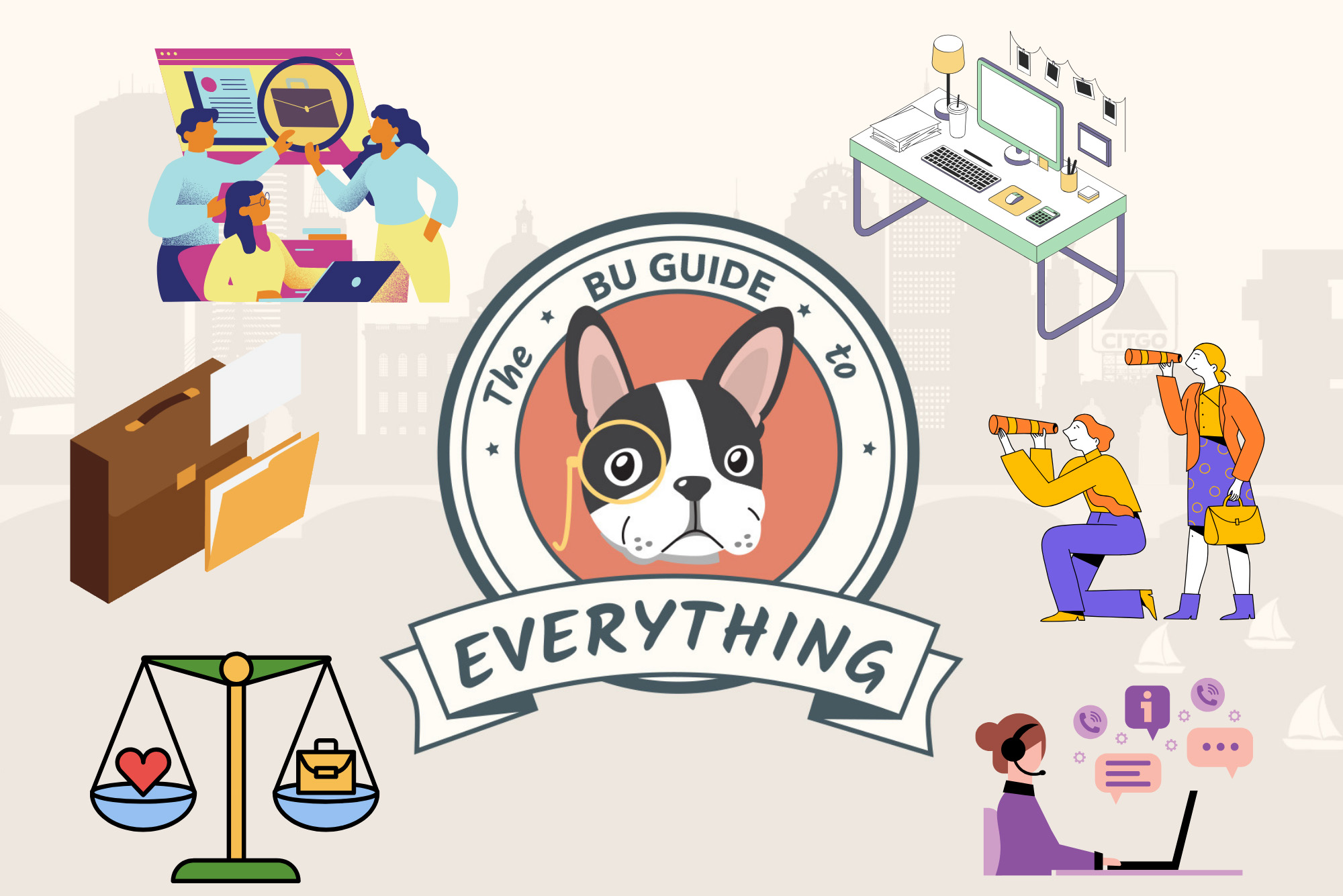The image appears to be a vibrant and colorful digital advertisement or book cover for something called "The BU Guide to Everything." Dominating the focus is a circular logo with the text "The BU Guide to Everything" encircling it. Inside the circle, there is a pink background that highlights the head of a Boston Terrier, appearing almost pug-like, wearing a yellow monocle on its left eye. Below the dog's face, a ribbon banner reads "everything."

Surrounding this central image are various 2D cartoon drawings representing different themes. To the top left, an office scene shows three people looking at a projection screen, with a briefcase below them. The top right features a detailed workspace complete with a keyboard, monitor, lamp, drink, file folder, calculator, mouse pad, mouse, and pens, with sticky notes and a picture on the wall.

In the middle left area, a briefcase, manila folder, and a piece of paper that appears to be pulled out of the folder are depicted. Opposite this, to the right, two individuals—a male kneeling and a female standing behind him—are looking through devices resembling periscopes or telescopes towards the central dog image. Below them, a woman wearing a headset typifies a call center agent, seen typing on a laptop with multiple thought bubbles featuring ellipses and a phone. Lastly, at the bottom left, a balancing scale contrasts a heart on one side and a briefcase on the other, symbolizing balance between work and personal life.